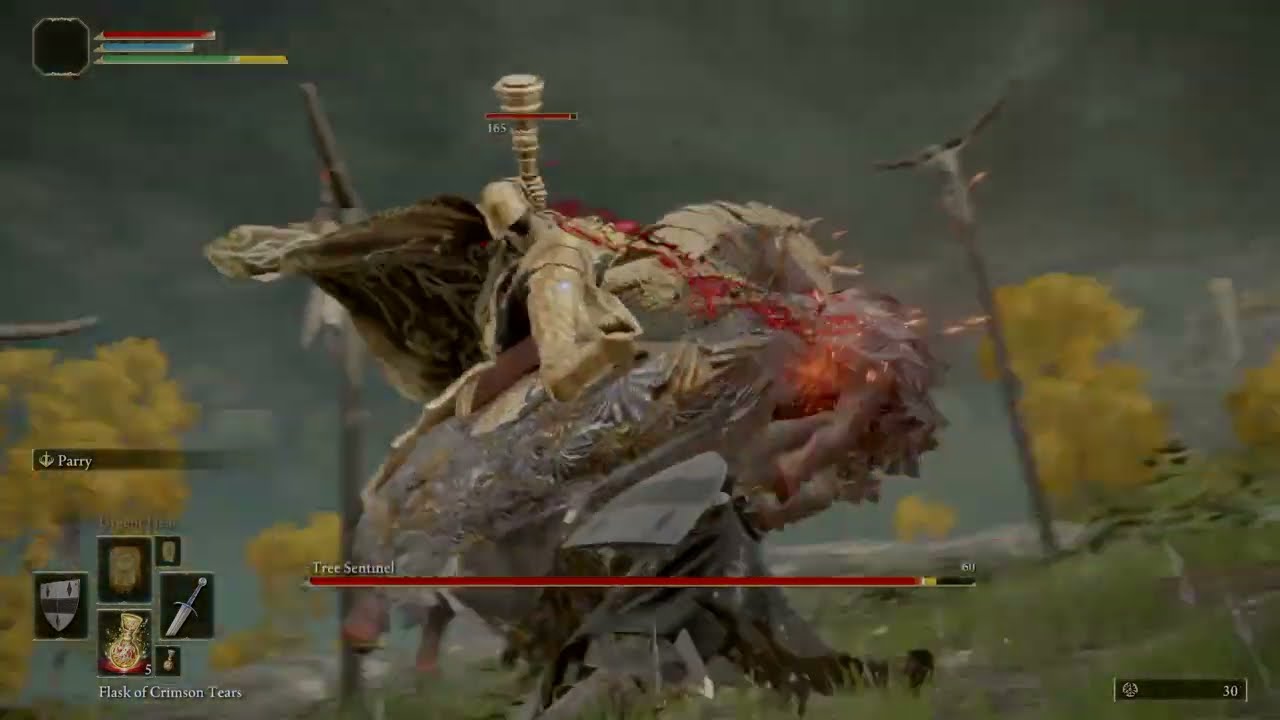The screenshot is from a third-person video game depicting an intense battle between the player character and a monstrous creature called "Tree Sentinel." The scene is dynamic, with various elements in motion. The Tree Sentinel is situated in the center of the image, appearing as a beige and brown disfigured beast with long legs. There is a dramatic burst of orange in the middle, which might be blood and other materials flying out from the creature, suggesting it has just been struck by an attack.

Above the creature, there’s a gold-colored health bar for the player character, showing a mostly full status marked with the number "165." In stark contrast, the Tree Sentinel’s health bar spans the bottom of the screen, appearing mostly red but transitioning to yellow and black towards the right end, with the number "611" nearby indicating its remaining health.

The upper left corner of the screen features a gray box with three colored lines - red, blue, and green with a yellow tip - alongside additional interface elements such as a gray "Perry" bar with an anchor and several weapon and shield icons. In the bottom left corner, inventory slots are visible, including one marked "Flask of Crimson Tears." Meanwhile, the bottom right corner displays a black bar with the number "30."

The background sets a foreboding scene with a solid gray sky filled with heavy, dark clouds, and a grassy green terrain. A unique structure, resembling a tilted power pole, appears towards the right, with what could be yellow leaves or a burst of yellow smoke, enhancing the chaotic atmosphere of the battle.